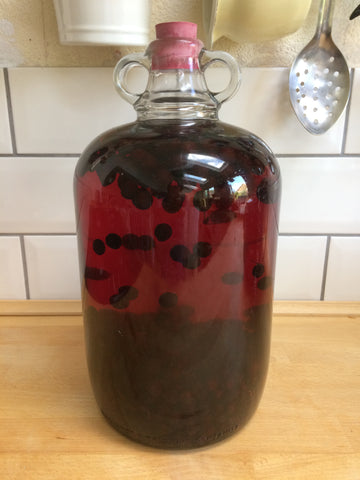The picture captures a detailed scene in a well-lit kitchen. At the center of the image is a tall, fat clear glass jug featuring two handles near its top and sealed with a red cork. Inside the jug is a translucent red liquid, peppered with what appear to be dark purple berries or possibly cherries, some of which are floating and others settled at the bottom. This jug sits on a beige wood kitchen counter. The background is adorned with clean, white subway tile backsplash. Above the countertop, on the wall, hang several kitchen utensils: a silver slotted spoon on the right, a yellow bowl in the middle, and a white container partially cut off in the left corner. Additionally, the glass jug reflects sunlight streaming through skylights and windows, suggesting a sunny day with some clouds in the sky.